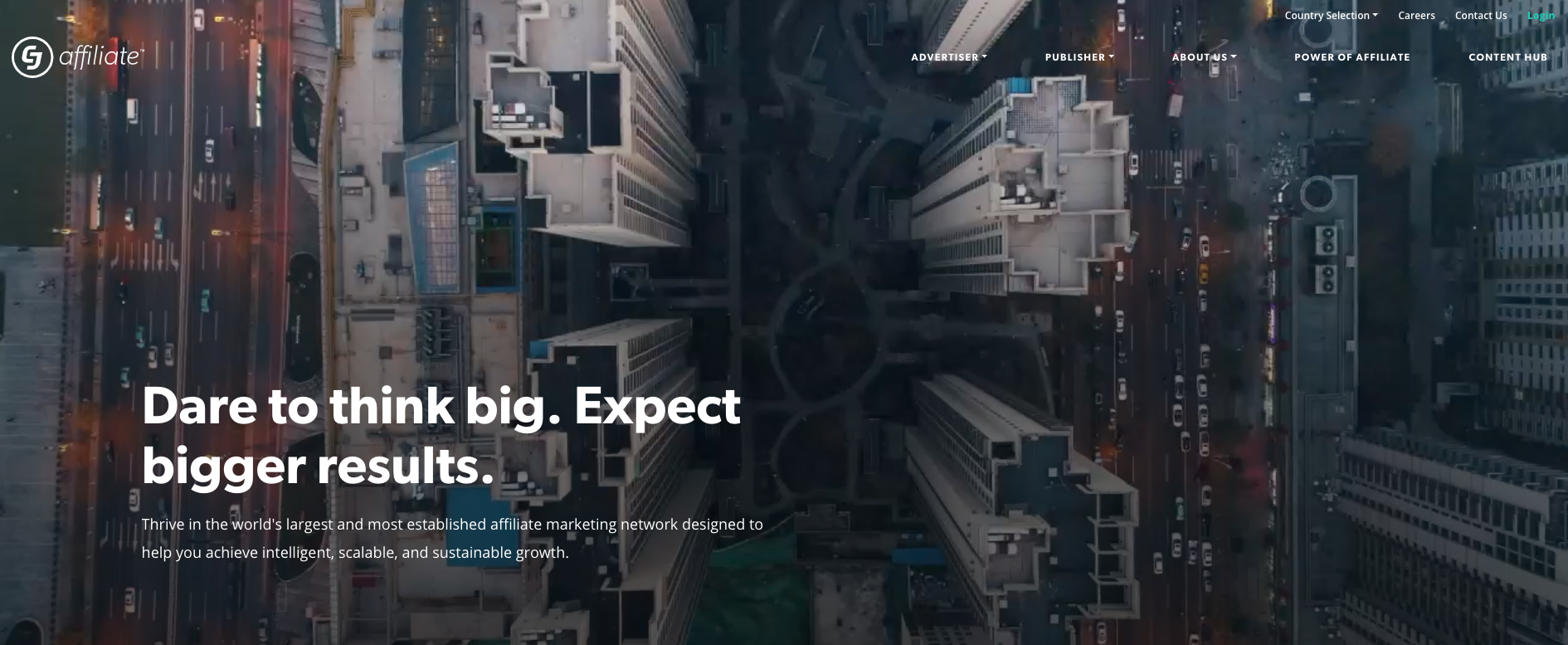A screenshot of a webpage is depicted in the image. In the top left corner, there is a logo which appears to read "CJ" followed by the word "Affiliate." The precise text within the logo is somewhat unclear. The top right corner contains a menu with five clickable sections, though the text is too small to decipher. In the lower left corner, bold white letters proclaim the motivational phrase, "Dare to think big, expect bigger results." Below this, there is additional text that is too small to read.

Dominating the left side of the image is a freeway that undulates up and down, carrying cars in both directions. Flanking the freeway are various buildings, and at the center lies a courtyard-like area. This courtyard features winding paths that intricately circle around each other, creating a spiraled layout. Surrounding this courtyard, tall buildings, possibly apartment complexes, rise on both sides. To the right, another road stretches vertically across the image, bustling with heavy traffic on both sides, highlighting significant congestion.